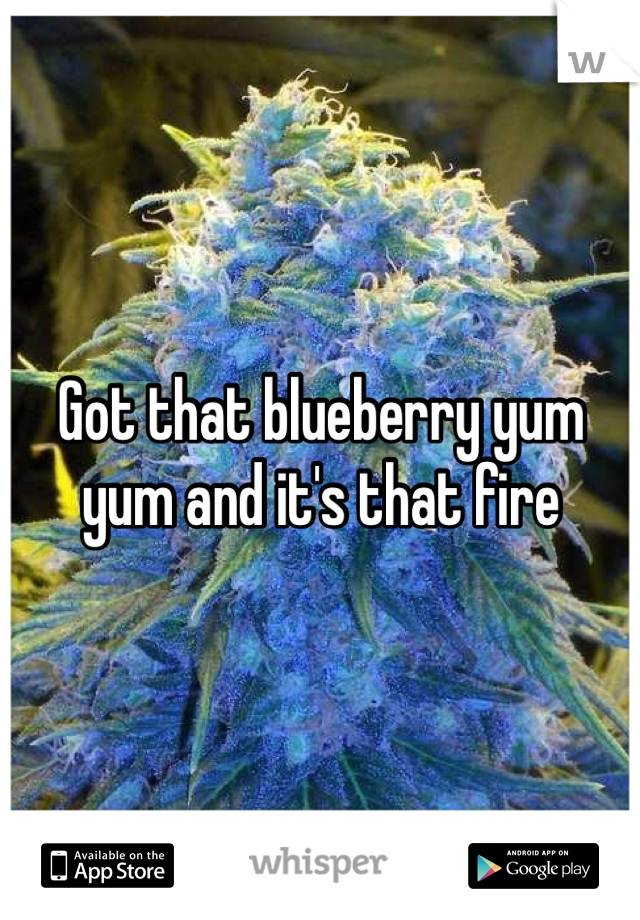The image predominantly showcases a plant-like object resembling algae, commonly identified as weed, which fills the majority of the frame. This central object is hairy, with a mix of blue, white, and green hues, and has a pointed top with rounded sides that expand outward as it descends. The backdrop features blurred green leaves, possibly from a palm tree, against a dark green and black background, suggesting an outdoor or grow house setting.

Overlaying the image is a prominent white text in bold letters with a black outline, reading "got that blueberry yum-yum and it's that fire," positioned in the middle. Additional text at the bottom of the image advertises various platforms: "available on the App Store," "Whisper" in gray lowercase letters at the center, and "available on Google Play," along with its logo, on the right-hand side.